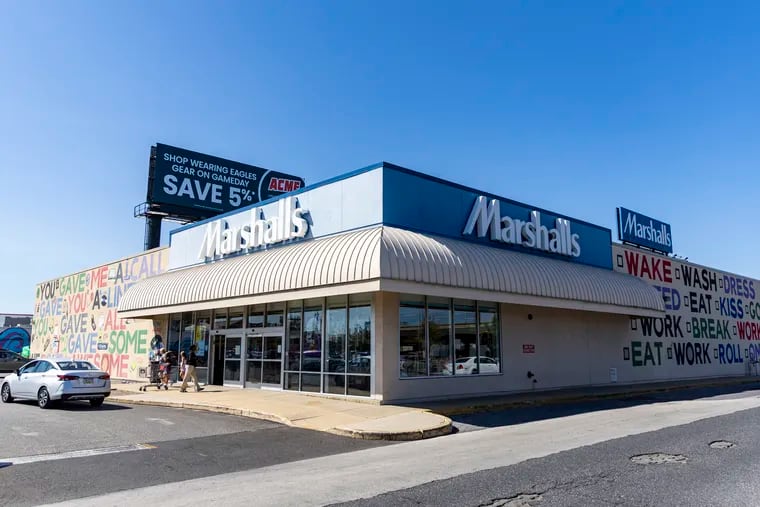The image captures a corner view of a Marshalls retail store set in an outdoor, daytime environment with a blue sky. The store, identifiable by its blue sign with white lettering that reads "Marshalls" on both sides, features large glass windows and doors beneath an awning. On the right-hand side of the building, large colorful words such as "wake, wash, dress, eat, kiss, work, break" are prominently displayed in various shades including red, black, blue, and green. Similarly, on the side where a white car is parked, words like "give me a call, give, all gave some" are painted, though some text is obscured by the vehicle. Behind the building, a sizable dark blue billboard with white lettering promotes shopping in Eagles gear on game day to save 5%. A few people are seen walking towards the entrance, providing a lively touch to the street scene, which appears to be captured from an angle slightly out in the middle of the street.